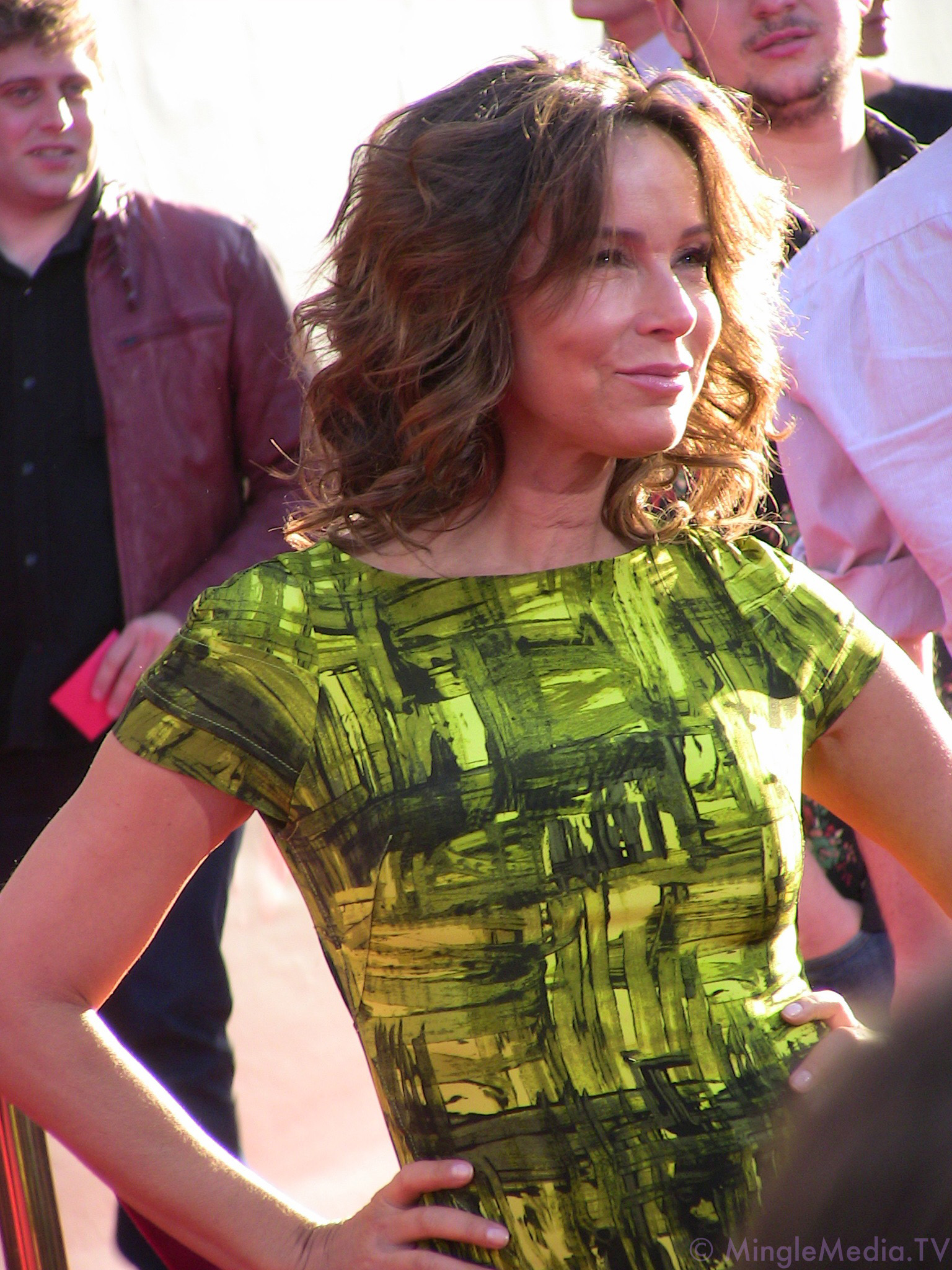In the image, the main focus is a woman standing at an event amidst a crowd. She has her hands on her hips, elbows bent at a 90-degree angle, and she is looking off to the right with a slight smile on her face. Her wavy, curly brown hair falls to about shoulder-length. She is dressed in a distinctive short-sleeved green dress, adorned with black smears resembling paintbrush strokes or a modern cubist art print. 

The bright sunlight illuminates the scene, casting light on her and the surrounding individuals. In the background, there are several figures, including a man in a black button-down shirt and a brown leather coat holding a red item, possibly a piece of paper or a phone case. Additionally, a man's face with a goatee and mustache is partially visible in the upper right corner of the image. Another person's white shirt can be seen behind the woman on the right side. In the bottom right corner, the logo "minglemedia.tv" is visible, including a possible copyright symbol. The crowd behind the woman appears to be smiling or looking in her direction, contributing to a lively and engaging scene.